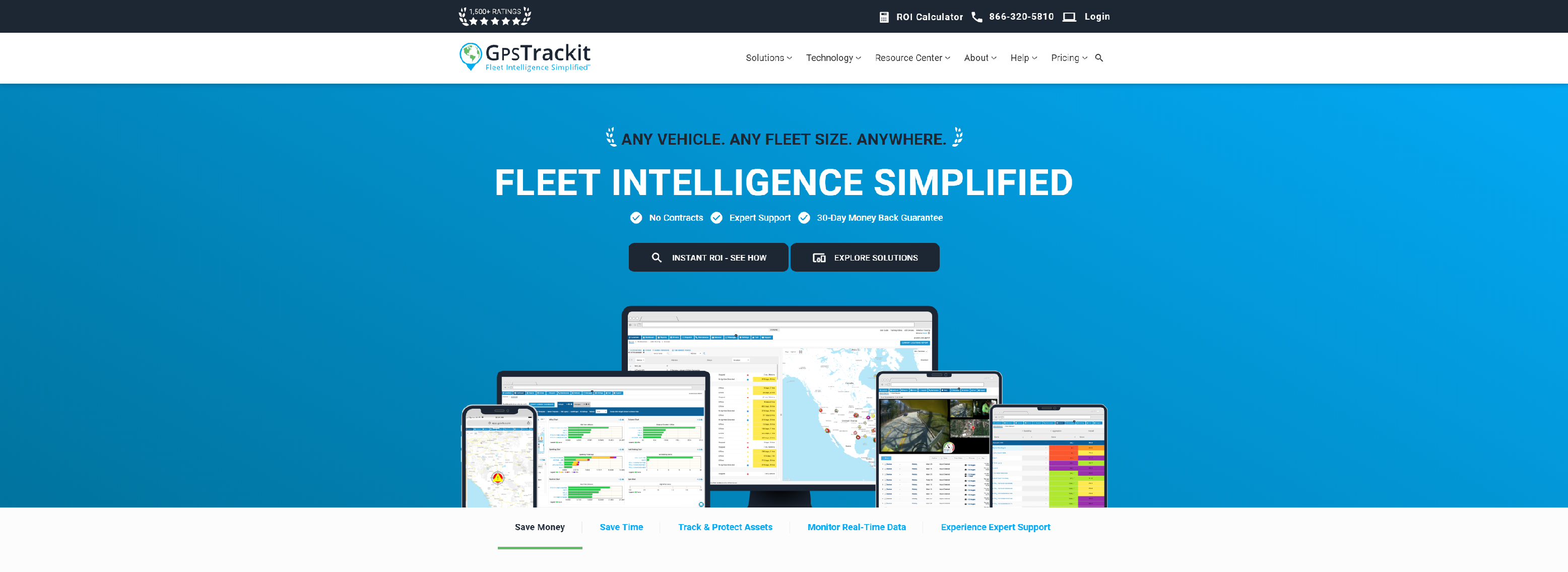The image features a detailed header section with a black bar, adorned with a stylized, curling leaf design flanking both sides. Centered within the bar are five white stars. Above the stars, there is unidentifiable text. To the right of this section, there's an icon followed by several words, which include a telephone icon and presumably a telephone number, then another icon, possibly indicating a login option.

Below this header is a globe icon accompanied by the text "GPS Track It," with an additional line of blue text beneath it that is unreadable. This is followed by six navigational tabs, the labels of which are not discernible, concluding with a magnifying glass icon on the far right, likely indicating a search function.

Central to the image is a prominent blue box containing visuals of a mobile screen, a computer screen, a couple of tablets, and various computer screens, all intertwined with leaf motifs. The box displays the message "Any vehicle, any fleet size, anywhere" and the slogan "Fleet Intelligence Simplified" in bold white letters.

Beneath this main visual area, three horizontal bullet points are listed, though their content is not readable. Subsequently, there are two black rectangles, the first of which resembles a search bar, while the function of the second remains unclear.

At the bottom part of the image, there are five selectable options, with the leftmost option distinctly underlined in green, signifying it as the current selection.